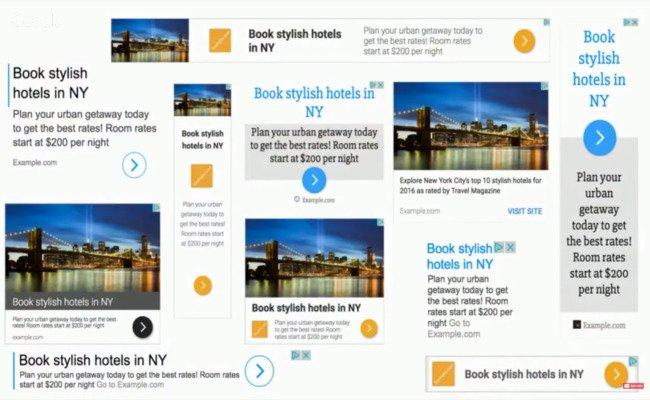The screenshot depicts a segment of a website, lacking the identifiable header and footer typically seen on web pages. The layout is reminiscent of a newspaper, featuring sections of content arranged in a combination of multiple columns and rows. Prominently, the same image is repeated throughout the segment: a striking suspension bridge, likely connecting to New York City, given the context.

The bridge image, characterized by its suspension wires converging at the center, dominates the visual space. Surrounding this image, various text blocks provide information. Large text prominently promotes New York City's top 100 stylish hotels, urging viewers to "Book stylish hotels in NY" — a phrase that appears multiple times across the screenshot.

Additionally, there are calls to action such as "Plan your urban getaway today to get the best rates," with a note indicating that room rates start at $200 per night. The repetition of different banners and promotional texts suggests that they are consolidated into a singular page layout, creating an impression that they might originally have been intended as separate elements. This dense arrangement of visual and textual content aims to entice visitors to explore stylish hotel options for a sophisticated stay in New York City.